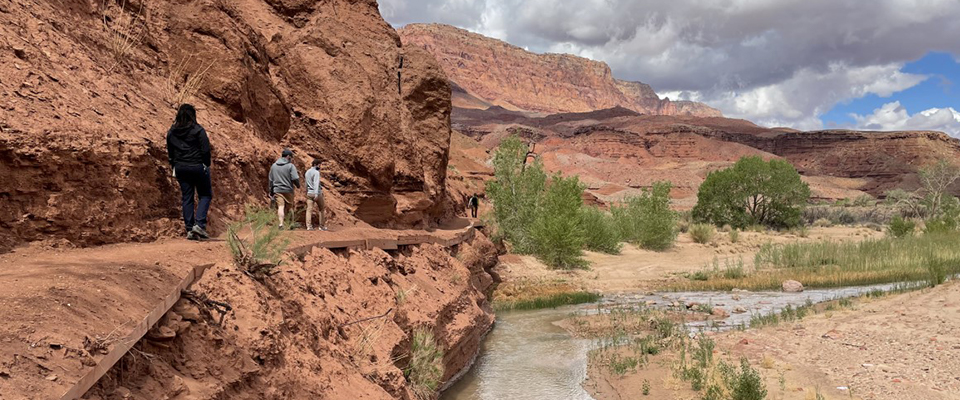In this rectangular photograph with landscape orientation, the viewer is presented with a scenic outdoor path carved into a red stone cliffside. The central focal point is a small creek with brown water, adorned with sandbars, and flanked by large white boulders on either side. Above the creek's sandy bank, lush green strands of grass are interspersed, leading to a sandy slope.

To the left of the creek, the red cliff showcases a pedestrian walkway that has been hewn into the rock, providing a flat path. Three individuals are seen walking on this path, all with their backs to the camera: one wears a black hoodie with black pants, another sports a gray hoodie with tan shorts, and the third person dons a blue long-sleeve shirt. Further along this path, a fourth person is visible in the distance, also with their back to the camera.

In the background, the scene is framed by additional orange rock cliffs and pockets of tree foliage, with a mostly cloudy sky, offering occasional glimpses of blue. The photograph beautifully captures the interplay between the rugged terrain and meandering creek, enriched by the human elements traversing the dramatic landscape.